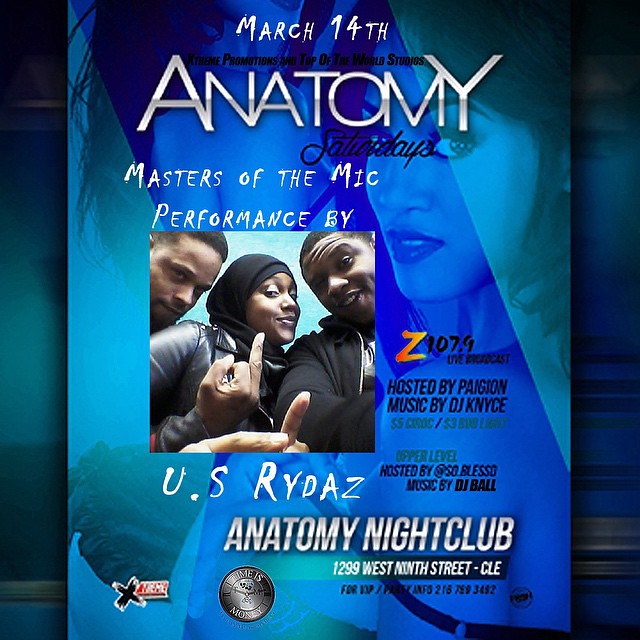This is a detailed flyer for the Anatomy Nightclub's "Masters of the Mic" event on March 14th. The flyer predominantly features hues of blue and turquoise. The background showcases an image of a woman, overlaid with event details in white text. Central to the flyer is a photograph of three young African-American artists – one woman and two men – with two of them making irreverent gestures. Highlighted in yellow, the flyer announces a live broadcast by Z107.9, hosted by Page and featuring music by DJ Nice. Additional entertainment will be provided by DJ Ball on the upper level, hosted by So Blessed. The flyer also advertises drink specials: $5 for Ciroc and $3 for Bud Light. At the bottom, the venue’s address is listed: Anatomy Nightclub, 1299 West 9th Street, with a phone number for VIP reservations.